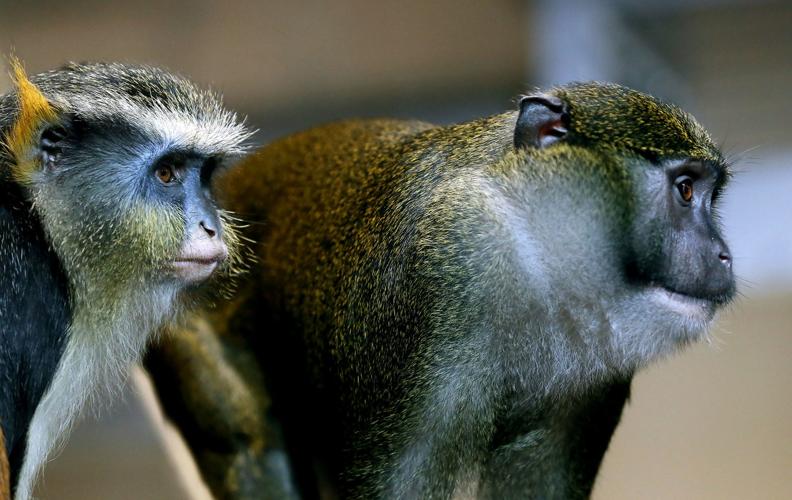The image depicts a close-up side view of two monkeys or baboons gazing intently to the right. The larger monkey on the right, with a serious and somewhat wistful expression, has a greenish-brown coat. Its face is adorned with black leathery skin that extends across its forehead, down the nose, and around the ears, continuing under the bottom lip to the chest, where it meets patches of white fur. This monkey has black leathery ears and dark brown eyes, framed by a few whiskers.

Next to it, the smaller monkey exhibits similar coloration but has distinct differences in facial features. It showcases a narrower, pinkish nose with bluish fur around the eyes, and its face is not entirely leathery but only in parts. This monkey's white fur highlights its eyebrows, running as long strands of hair, with a patch of pointed orange hairs above its ears extending down to its neck, adding a contrast to the overall appearance. It also has yellowish fur around its ears and greenish-yellow cheeks, with a darker gray body partially visible.

Both animals share a background that is completely out of focus, enhancing the clarity and detail of their features. They appear moderately sized, potentially regular tree monkeys, though their specific breed is unidentified. The image captures their attentive gaze, as they fixate on something unseen off to the right, their expressions adding an air of solemnity to the scene.